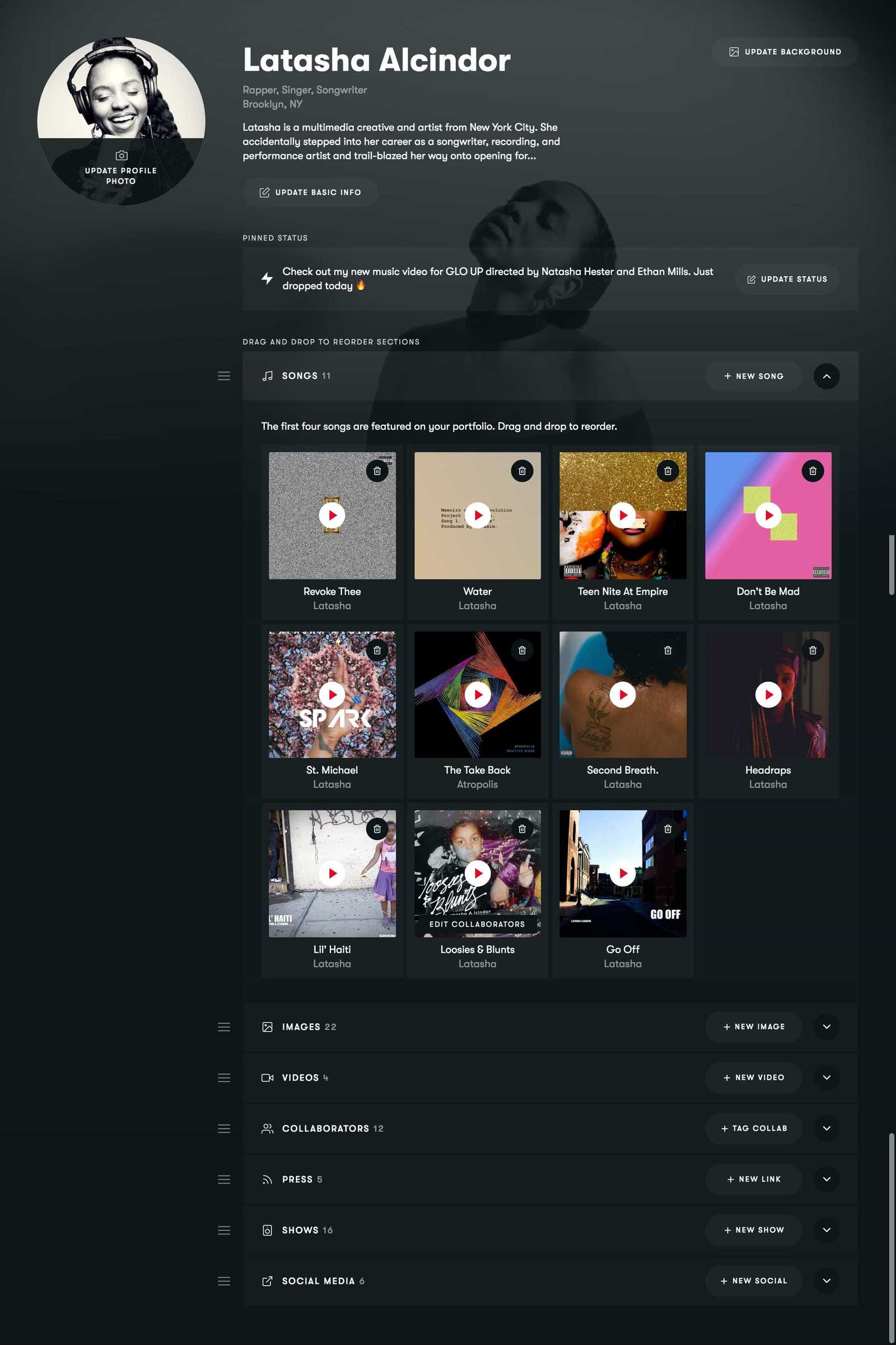This screenshot captures the profile page of LaTosha Alcindor, prominently displayed at the top. To the left is a prominent circular profile picture featuring a black woman with long braided hair. The lower half of this circle is darkened with the text "Update Profile Photo."

Below her name, the profile identifies her as a "Rapper, Singer, Songwriter" from Brooklyn, New York. 

The page further includes a bio section under her identifiers, followed by an "Update Basic Info" button. Beneath this section, a pinned status area is visible, with a status bar and the option to "Update Status" located to the right.

The profile also showcases LaTosha's musical portfolio; a section labeled "Songs" features a "Plus New Song" button to the right. Displayed below this button are eleven songs arranged in three rows, each with a thumbnail image and a play button, allowing for immediate interaction and listening.